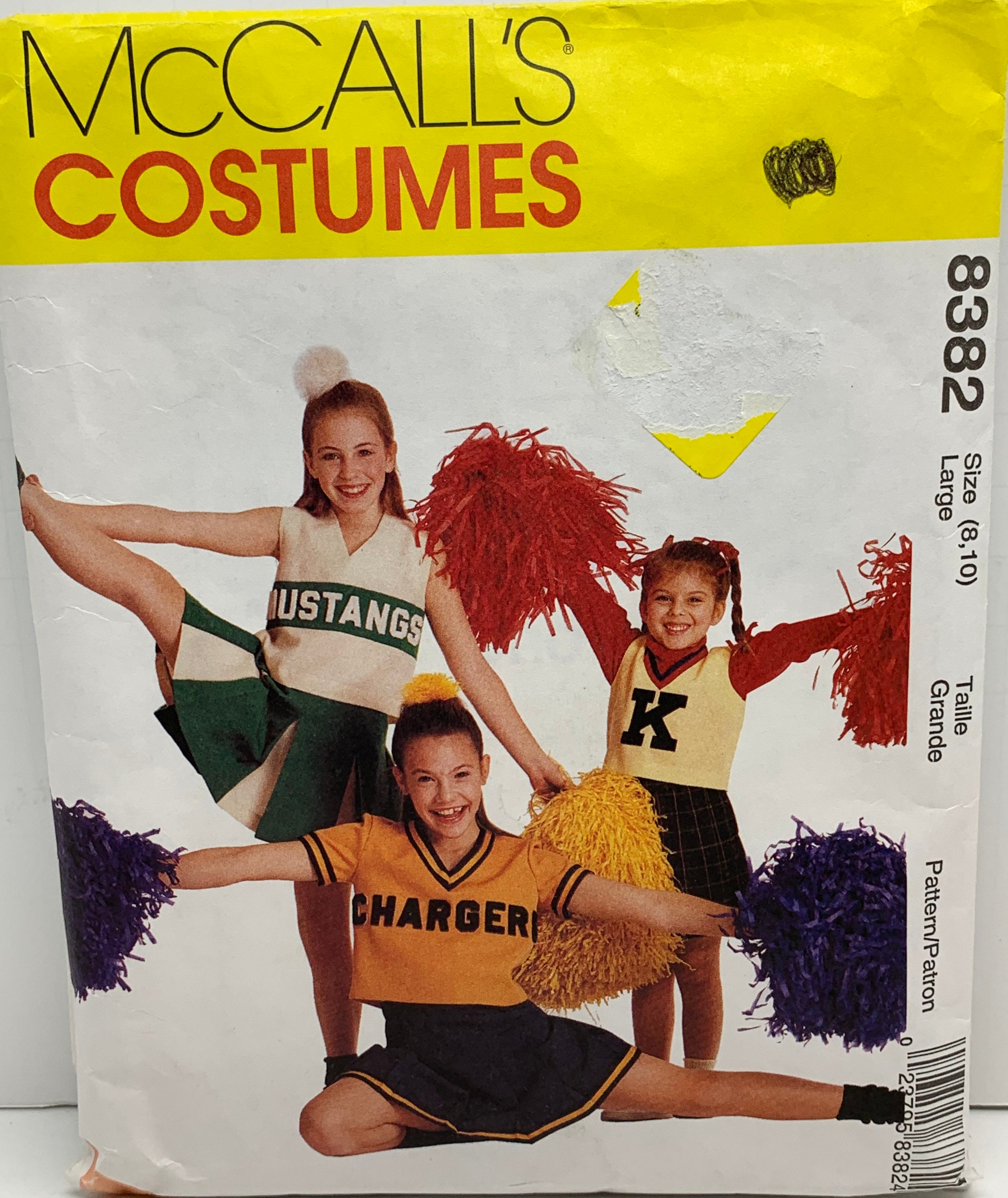This image is an advertisement poster for McCall’s Costumes, prominently featuring a yellow banner at the top with "McCall’s" in fine black text and "Costumes" in bold red text. The centerpiece of the poster showcases three young adolescent girls dressed in different cheerleader outfits, striking energetic cheer poses complete with pom-poms. On the left, one girl is exuberantly lifting her leg, donning a vibrant green and white Mustang's uniform with "Mustangs" emblazoned across her chest and a matching skirt. In the center, another girl sits confidently in a gold and black Chargers outfit, complete with a black skirt and black socks. The girl on the right, the shortest of the trio, wears a vest featuring a bold "K" over a red shirt, complemented by a matching striped skirt. The various aspects of the image suggest that McCall’s Costumes specializes in providing a variety of cheerleader uniforms, and possibly other sports attire, highlighted by the detailed and dynamic presentation of each cheerleader outfit.